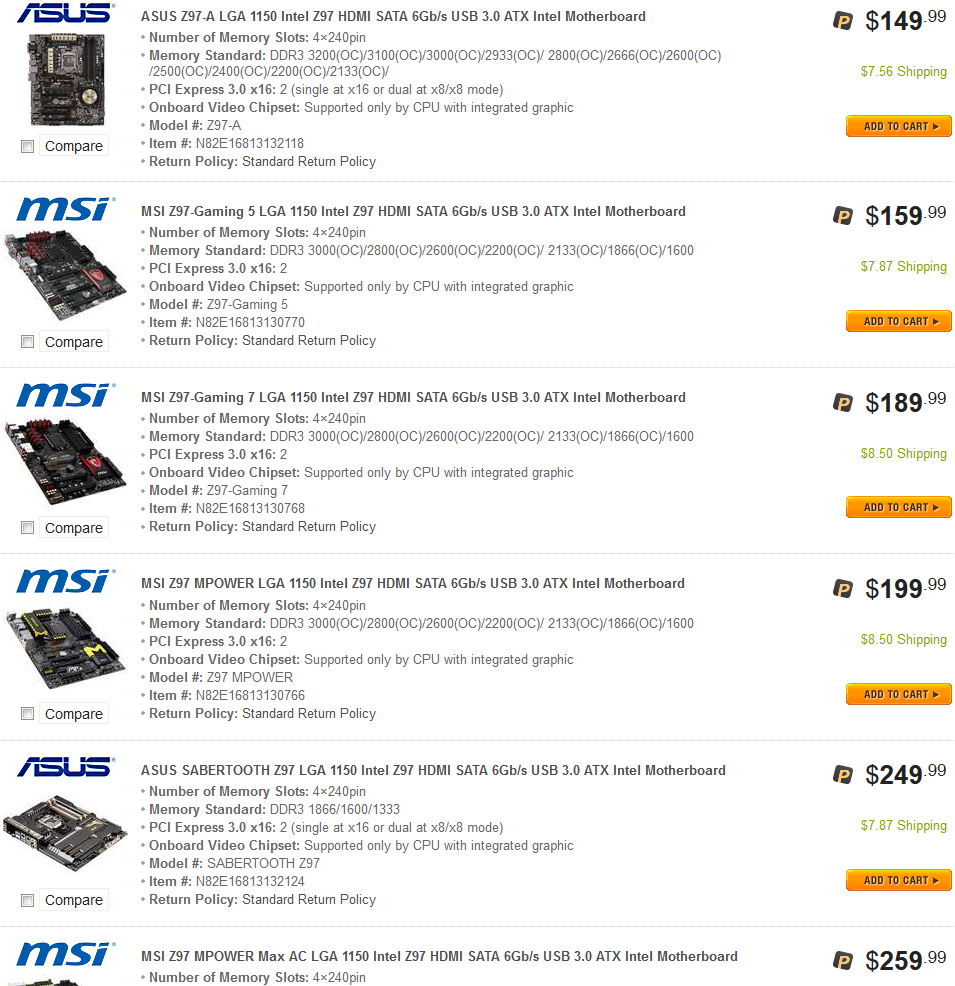The screenshot features a list of various ASUS and MSI motherboards, organized in a comparison format. On the left side, there are truncated images of at least five motherboards from both ASUS and MSI. The sequence appears as ASUS, MSI, MSI, MSI, ASUS, and MSI again. Each motherboard image has a square button labeled "Compare" beside it.

To the right of the images, detailed descriptions of each motherboard are provided. These descriptions include specs such as the number of memory slots, memory standards, PCI Express details, onboard video options, chipset type, model numbers, item numbers, and return policy. The specifics vary across different models.

Prices for the motherboards are listed on the far right, ranging from $149 to $259, in black text accompanied by a "P" icon to the left. Below each price, the estimated shipping cost is indicated in green text.

Each motherboard listing also features an orange "Add to Cart" button, with the text in black capital letters and an arrow pointing to the right.